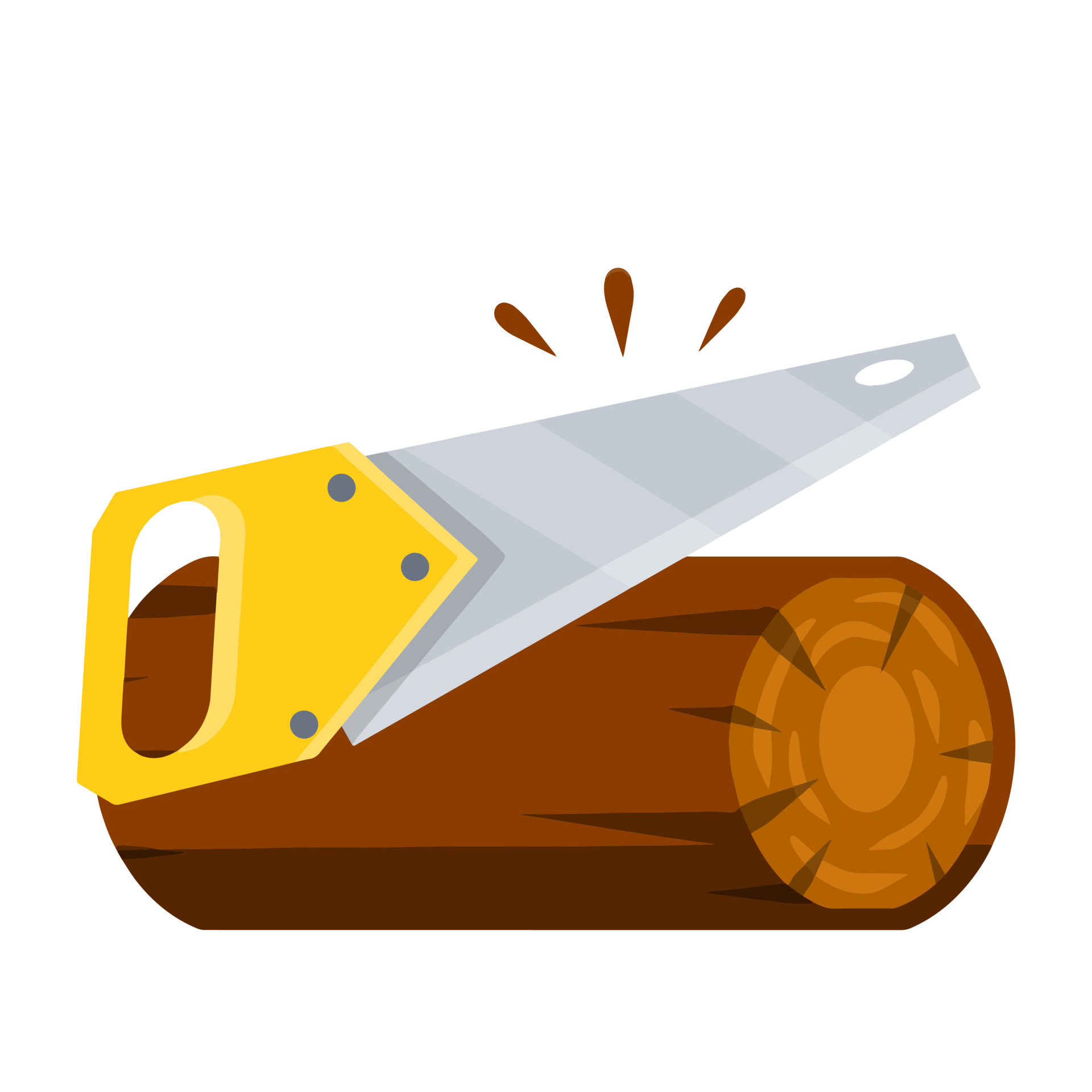This digital clip art illustration, set against a completely white background, features a log being sawed in half. The saw, with its smooth, beveled, gray metal blade and a yellow handle, is poised to cut through the symmetrical log. The blade exhibits a unique design, tapering from a wider handle end to a blunted flat tip, with an oval hole near the end and three screws securing the handle. The handle itself is spacious enough to fit all four fingers comfortably. The log, shown in a rich brown color with a lighter center, reveals intricate details including seven distinct cracks on the visible cut end and shading that adds depth. At the top of the image, three droplet-shaped wood chips float above the saw blade, indicating the action of sawing.